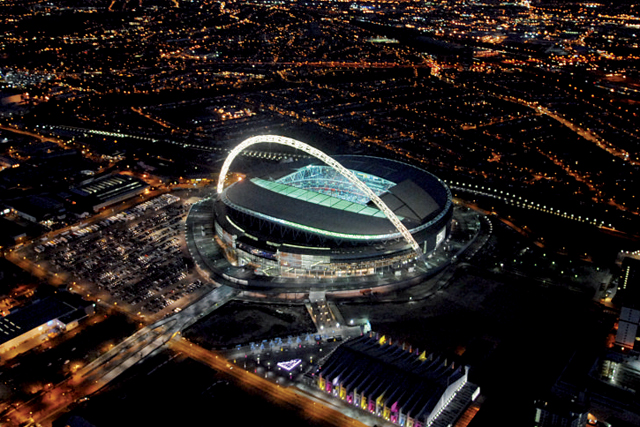Captured from a high aerial perspective, possibly from a blimp, this nighttime photograph showcases what appears to be Wembley Stadium, dazzling in its modern and intriguing design. The circular stadium, featuring an open roof, is enveloped in brilliant white lighting that starkly contrasts with the warmer, orange hues of the surrounding cityscape. A distinctive illuminated arch, reminiscent of a giant LED-lit handle, spans majestically across the stadium's top, making it a prominent beacon in the night. The parking lots teeming with cars and the lively atmosphere suggest an ongoing event, with vibrant activity spilling from the stands into the bustling city beyond. The bright stadium lights illuminate the structure with an impressive glow, asserting its importance as the centerpiece of this vivid and dynamic nocturnal scene.